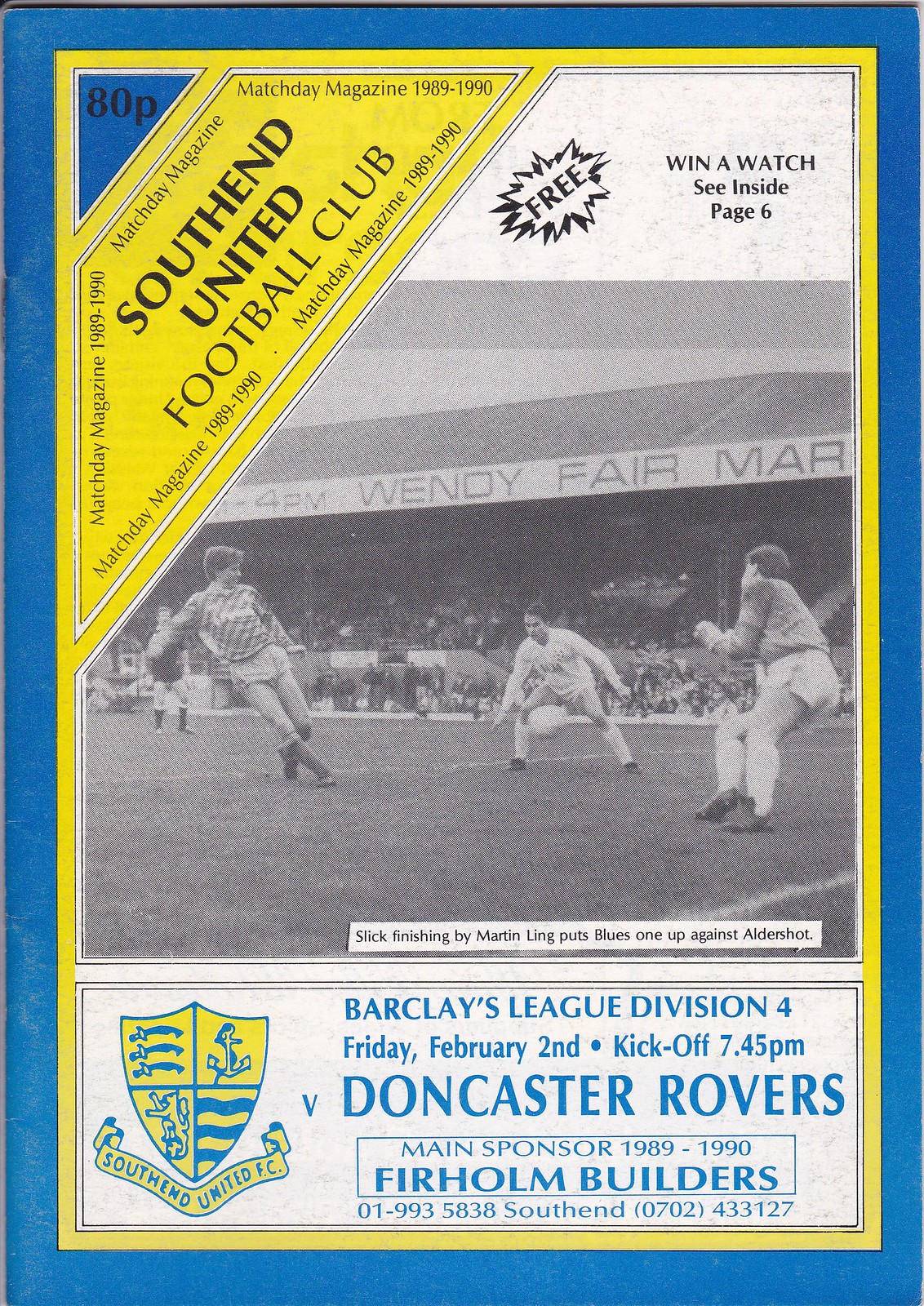This is a matchday program cover for South End United Football Club from the 1989-1990 season. The cover is bordered with a blue outline followed by a yellow outline. In the top right-hand corner, there is a blue triangle with "ADP" written in black text. Below that, in black block capitals, it states "South End United Football Club" and repeats "Matchday Magazine 1989-1990."

The center of the cover features a black and white photograph of men playing soccer on a pitch with a crowd in the background. Over the photo, it says "FREE" at the top, and "Win a watch - see inside page 6" on the right-hand side. At the bottom right of the image, a caption reads, "Slick finishing by Martin Ling puts Blues 1 up against Aldershot."

At the bottom of the cover, there is a yellow and blue crest on the left that says "South End United FC." Adjacent to this, in blue text on a white background, it reads, "Barclays League Division 4, Friday, February 2nd, Kickoff 7.45 PM vs Doncaster Rovers." Below this, it mentions the main sponsor for 1989-1990, Firholme Builders, along with their addresses and phone numbers: "01-993 5838" and "(0702) 433 127."